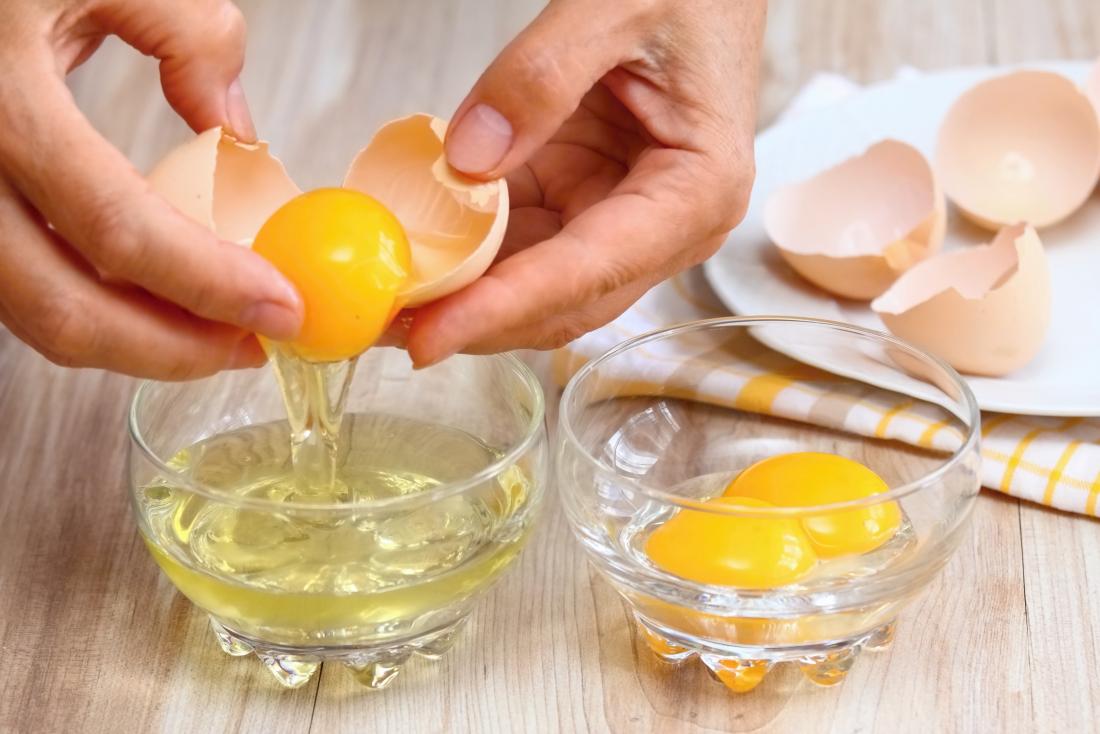This photograph captures a close-up, zoomed-in view of a pair of presumably Caucasian hands in the process of cracking an egg over a pair of small, clear glass bowls resting on a light wooden surface. The hands are positioned to separate the egg whites from the yolk, with one of the bowls receiving the whites while the yolk remains partly within the eggshell. To the right of this bowl, another identical clear glass bowl holds two vividly yellow yolks. On the left side of the scene, a white plate is visible, housing three halves of eggshells. This plate sits atop a white dish towel adorned with yellow and gray stripes. The meticulous separation of eggs, as indicated by the contents of the bowls, suggests a deliberate culinary preparation underway, though the exact dish remains a mystery.